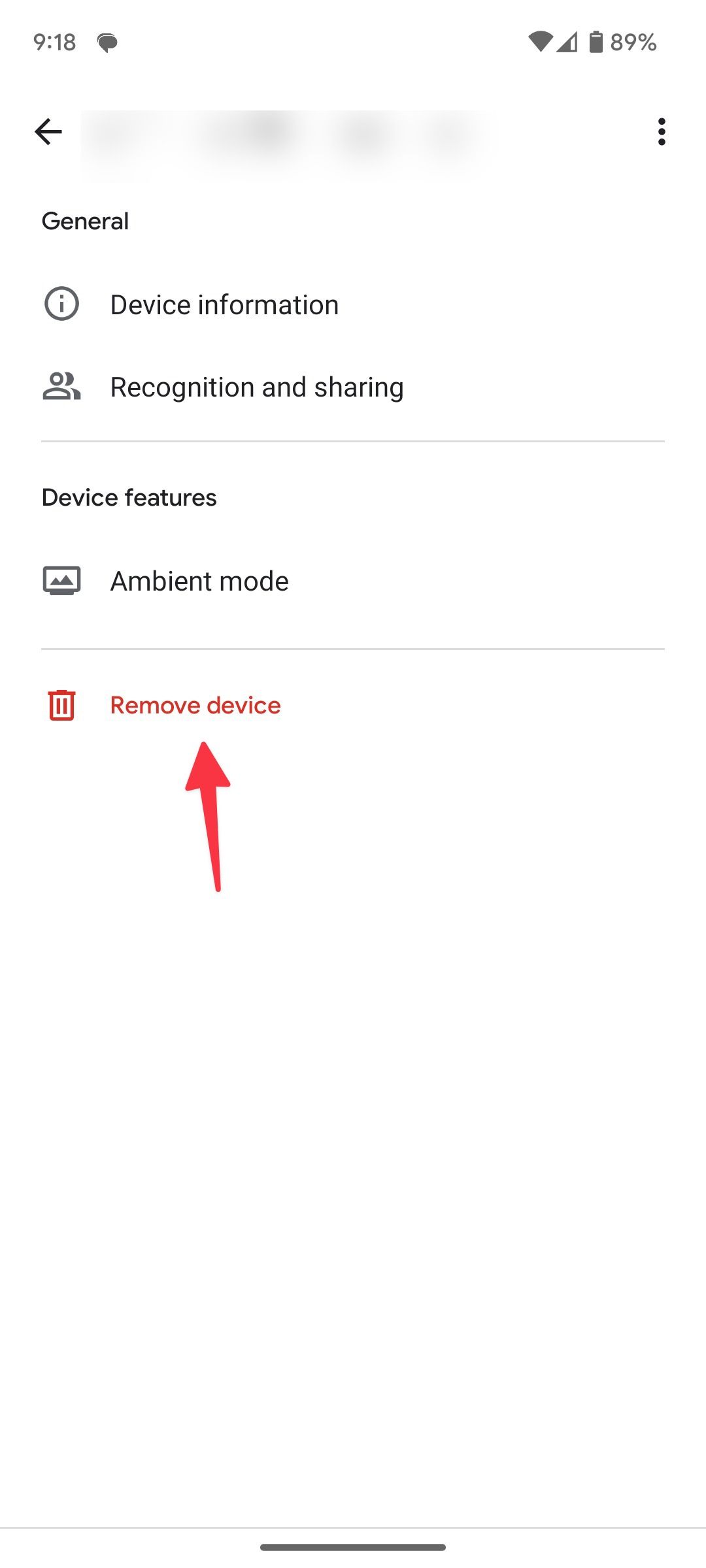A smartphone screenshot captured at 9:18 AM displays several interface elements. In the top right corner, the Wi-Fi signal icon is partially lit, indicating a moderate connection, alongside the battery icon showing 89% remaining charge. Directly below, an ombre-shaded navigation bar houses a back arrow on the left and a three-dot menu icon on the right.

The section labeled "General" appears prominently beneath this bar, accompanied by an information icon. Immediate subsequent options include "Device Information" and "Recognition and Sharing," each symbolized by relevant icons—a generic info symbol and an icon depicting two connected people, respectively.

A light gray separator line divides these options from the next section titled "Device Features." This section highlights "Ambient Mode," represented by a computer monitor icon, suggesting customizable display settings. Another gray spacer line precedes a red trash can icon linked to the bold text "Remove Device" with an accompanying large red arrow, indicating an option to delete or disconnect a device.